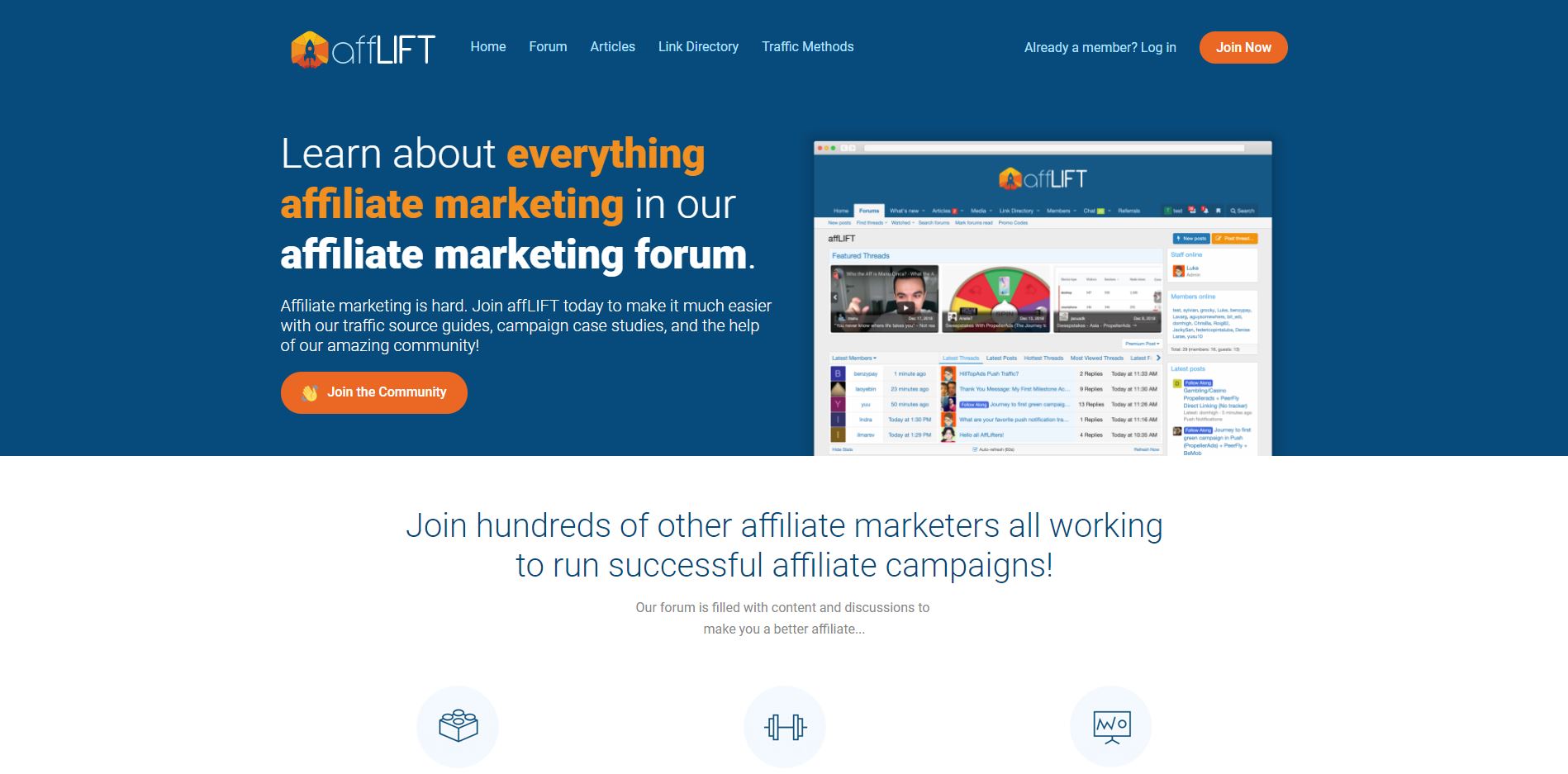This image depicts a screenshot of a web page with a large horizontally-oriented blue bar background that blends shades of navy and royal blue. Positioned at the top left corner is the brand name "AFLIFT," where "AFF" is in standard capitalization and "LIFT" is in all capital letters, alongside an icon featuring a rocket ship against a bright orange backdrop.

The top menu bar offers navigation options including "Home," "Forum," "Articles," "Link Directory," and "Traffic Methods." To the right side of the menu, there's a prompt for existing members to log in, along with an eye-catching orange button labeled "Join Now" in white text.

On the left side of the page, there's a bold statement: "Learn about everything affiliate marketing in our affiliate marketing forum." Here, "everything affiliate marketing" is highlighted in bold orange text, while "affiliate marketing forum" is in bold white, with the remaining text in standard white.

Continuing below, a message reads: "Affiliate marketing is hard, join AFLIFT today to make it much easier with our traffic source guides, campaign case studies, and the help of our amazing community." Underneath this is another prominent orange button that says "Join the Community."

Further down, another statement encourages visitors to "Join hundreds of other affiliate marketers all working to run successful affiliate campaigns." It notes that the forum is brimming with content and discussions designed to enhance affiliate marketing skills. The page concludes with a series of icons at the bottom.